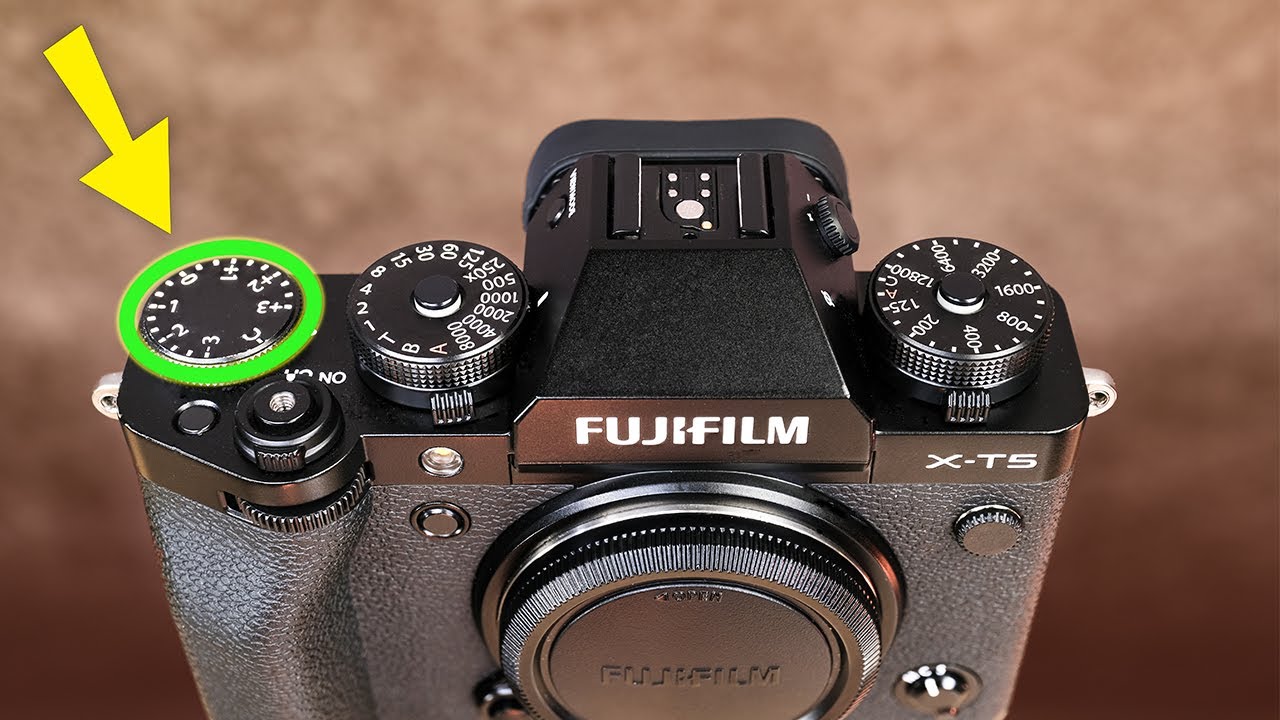The image showcases a Fujifilm X-T5 camera facing the viewer, highlighting the intricate details of its design. The camera boasts a textured black body with a metallic, smooth black top. It's equipped with a variety of features, including three dials on the top for different settings, with one of the dials encircled in green and highlighted by a yellow arrow, possibly indicating its importance or function, such as the exposure knob or shutter button. The lens on the front is protected by a cover, also branded with Fujifilm in white font, ensuring protection from scratches. The top middle section features a flash mount, and there are hoops on each side for attaching a carrying strap. The threaded button is also visible on top. The background is a blurred brown with a wood-like appearance, bringing a warm, rustic contrast to the sleek, modern lines of the camera.